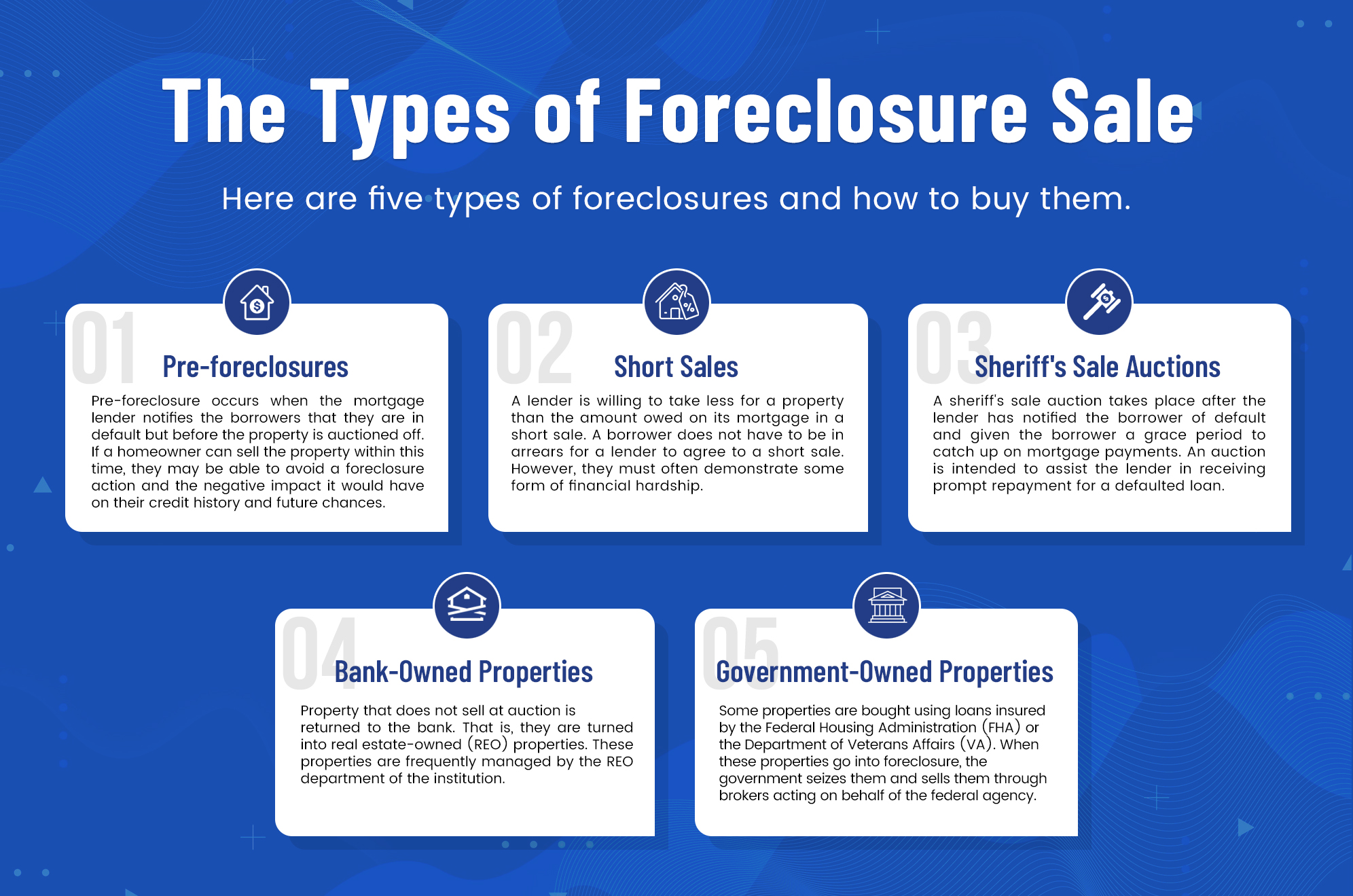The image features an informational slide with a blue background adorned with subtle, non-specific streaks and patterns. At the top, the white title text reads "The Types of Foreclosure Sale," followed by a smaller text subtitle: "Here are five types of foreclosures and how to buy them." The slide is divided into five sections, each numbered with gray numerals from 01 to 05, detailing different types of foreclosure sales. 

- **01: Pre-Foreclosures** - Identified by a house symbol with a dollar sign, this section explains that pre-foreclosure occurs when a mortgage lender notifies borrowers of default before the property is auctioned. Selling the property during this period can help homeowners avoid foreclosure and its negative impact on credit.
  
- **02: Short Sales** - Marked by a house with a price tag, this section describes short sales where a lender agrees to accept less than the owed mortgage amount. Borrowers must often demonstrate financial hardship, though they don't necessarily need to be in arrears.
  
- **03: Sheriff's Sale Auctions** - Illustrated with a gavel icon, this section details auctions that occur after borrowers are notified of default and given a grace period to make payments. These auctions help lenders receive prompt repayment for defaulted loans.
  
- **04: Bank-Owned Properties** - Featuring a house symbol that is either crossed off or roped up, this section covers properties that don't sell at auction and revert to the bank, becoming real estate-owned (REO) properties managed by the institution's REO department.
  
- **05: Government-Owned Properties** - Denoted by a column symbol with an indistinct feature on top, this section explains that properties bought with loans insured by the Federal Housing Administration (FHA) or the Department of Veterans Affairs (VA) are seized and sold by the government through brokers when foreclosed.

The overall structure includes three text sections on the top row and two on the bottom, each accompanied by blue icons to visually represent the type of foreclosure being described. The format is similar to a bank or financial institution slide designed to educate viewers about foreclosure sale types.